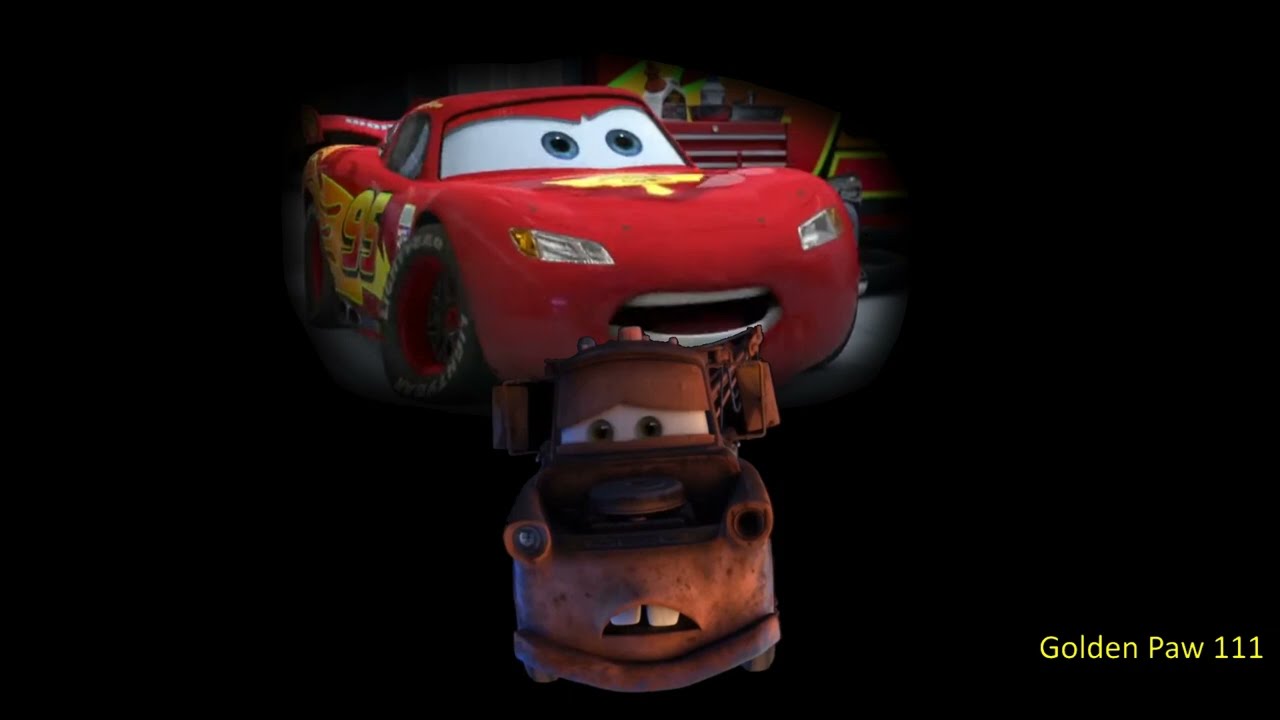The image depicts two animated cartoon cars from the Disney movie "Cars" against a pure black background. The bottom car resembles an old, rusted tow truck with dark gray or dark brown coloring. Its windshield forms sad, slanted green eyes underneath brow-like window visors, and its front grille features two white buck teeth, giving it a dog-like appearance. Stacked on top of this car is the iconic red Corvette-type NASCAR, Lightning McQueen, identifiable by its large white eyes with blue pupils. McQueen has yellow and orange flame-like markings on his hood and sides, accompanied by the yellow number 95 on the right passenger side. Notably, there is a yellow logo situated prominently on the same side. In the lower right-hand corner of the image, the text "Golden Paw 111" appears in yellow.